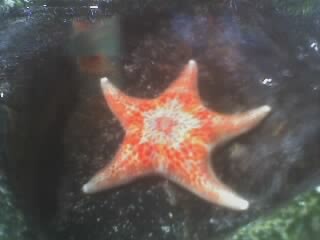This detailed photograph captures a starfish that appears slightly fuzzy or blurry, possibly due to being taken from behind glass, suggesting a zoo or aquarium setting. The image reveals a vibrant starfish with five points, vividly marked by bright white tips. The starfish's central section is predominantly orange, surrounded by a combination of white, yellow, and orange hues, forming intricate patterns. Notably, a light pink star shape radiates from the center, bordered by a lacy white star pattern, extending into the starfish’s arms adorned with dots of red, dark pink, and orange. The background, likely representing water, exhibits a marbleized blend of dark green, gray, blue, and white with lighter green shades in the bottom right corner. The starfish is positioned against dark, perhaps dark gray rocks, adding to the image's murky ambiance. The far left arm of the starfish is slightly curled, emphasizing its lively character.